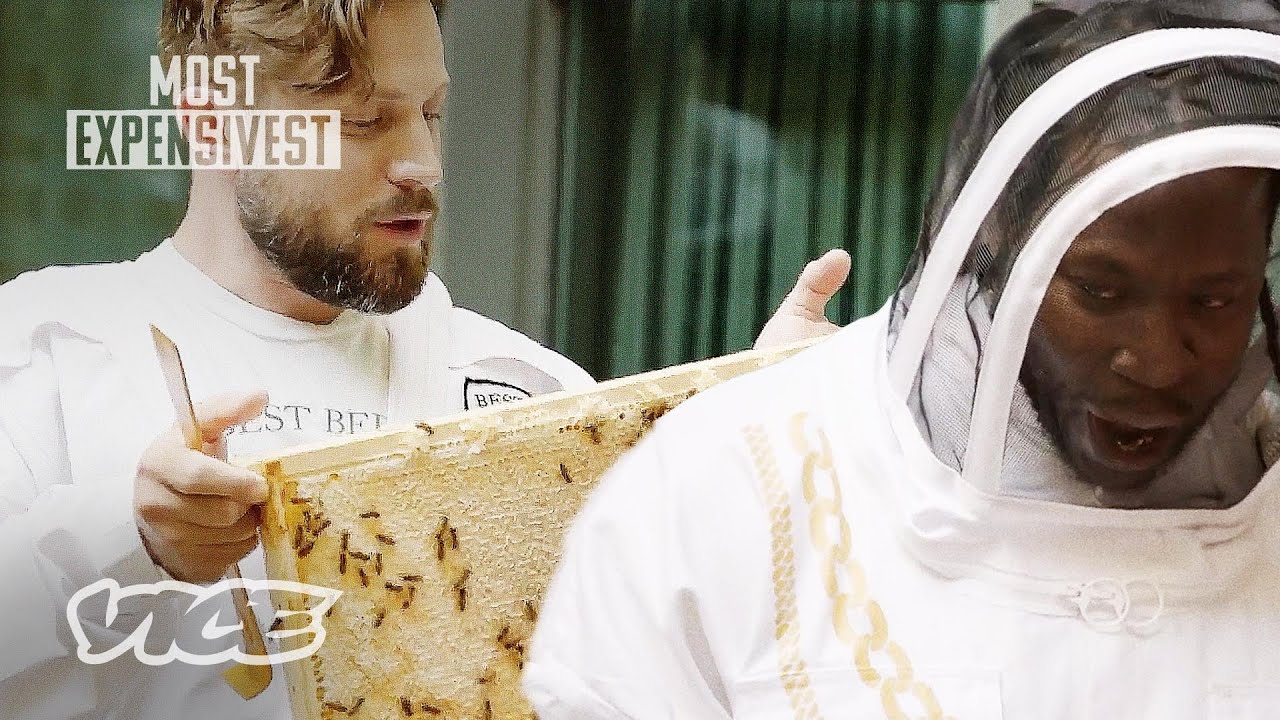The photograph features two bearded men dressed in beekeeping attire standing against a medium to light green background with vertical striations. In the upper left corner, the transparent text "Most Expensivest" is displayed, while the bottom left corner bears the Vice symbol. The man in the foreground, who is black, wears a white beekeeper suit complete with a mesh hood and a visible gold chain. He has an open-mouthed expression. Behind him stands a white man holding a rectangular bee frame, populated with bees and bits of honey, wearing a white shirt that appears to read "lost bet" or something similar. Both men seem focused on their task, with the white man looking intently at the bee frame. A green door is visible in the background.